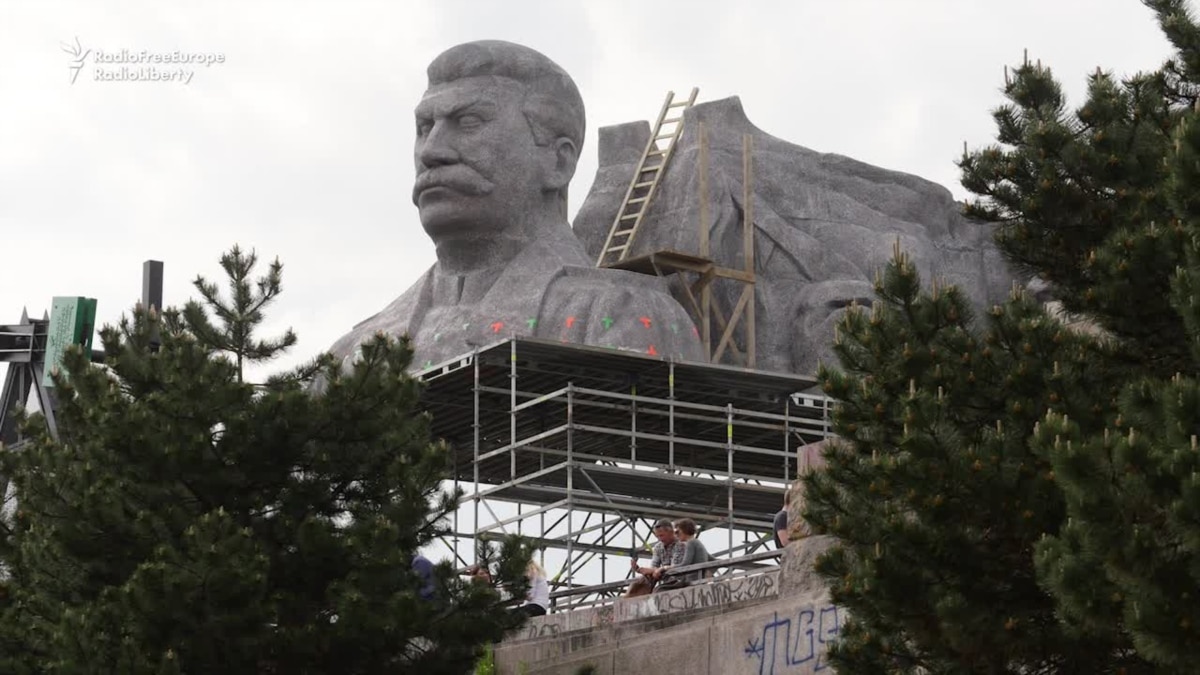In this outdoor daytime scene, a statue under construction dominates the center of the image, set against a cloudy, gray sky. The statue depicts a man with a large mustache, short hair, eyes closed, and wearing clothes with collars. The sculpture, which appears to be made of cement, is situated on a steel and iron scaffolding platform that extends horizontally across the image, adorned with railings, rods, and various levels. Behind the statue, there is a notable ladder and a large, rocky structure, possibly representing a mountain.

On the right-hand side of the image, a tall tree is visible, while a smaller tree can be seen on the left-hand side. Additionally, another tall structure rises behind the trees on the left. The foreground features people sitting and conversing beneath the scaffolding, next to a lower wall with inscriptions and graffiti. The left side of the image includes white lettering that reads "Radio Free Europe, Radio Liberty," along with a logo of a flame on a torch.